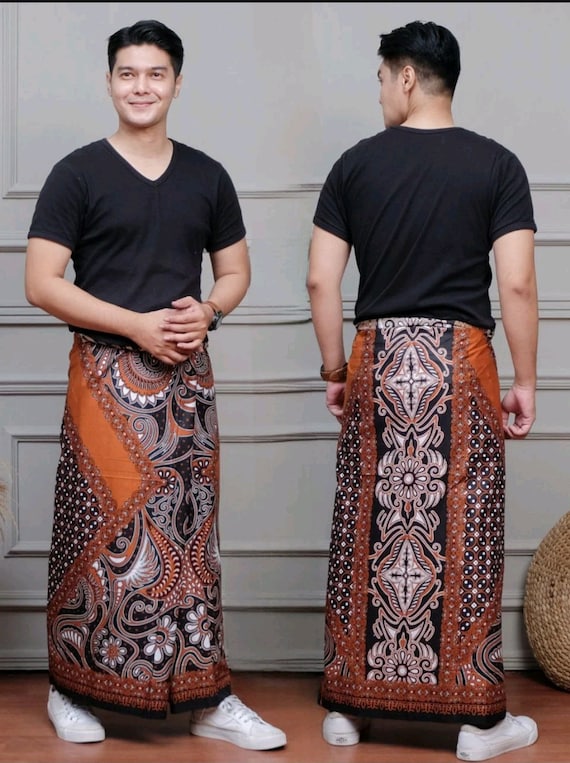The image is a photograph collage showcasing the front and back views of a light-skinned man with black hair, possibly of Asian descent, wearing a black v-neck t-shirt and an intricately patterned skirt. In the left photograph, the man stands facing the camera with a smile, hands clasped at his front. He is dressed in white tennis shoes and stands on a reddish hardwood floor. Behind him, the grey wall features various grey frames. The skirt, which falls to his shoes, is decorated with an array of designs including orange-circled diamonds, grey and orange fractal patterns, and a repeated intricate motif. On the right, the man is seen from the back, revealing a black rectangular design down the center of the skirt. His left wrist features a watch with a leather strap. His stance on both photos highlights the detailed patterns of the skirt and adds dimension to his outfit.